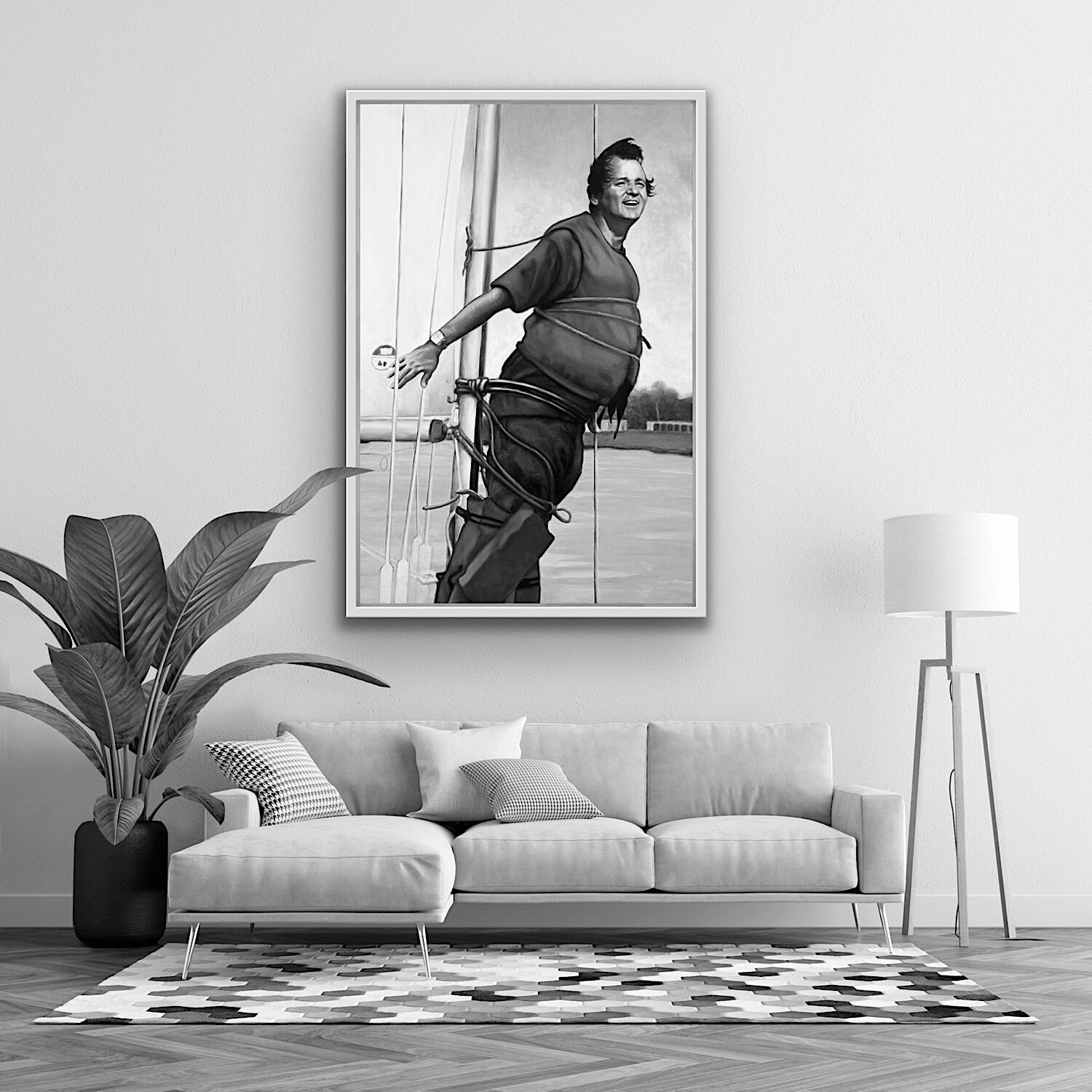The black and white product photograph showcases a staged modern living room with a distinct focus on a framed piece of artwork. The artwork features an illustration that appears to be edited post-production, depicting a man, likely a famous Hollywood actor, who has tied himself with dark ropes to a sleek metal sail of a sailboat. The background of the artwork hints at a picturesque shoreline with trees, houses, and a sandy beach. Below this eye-catching piece, a gray L-shaped corner couch occupies the center of the scene, accompanied by a large plant on the left and a lamp on the right. The couch features multiple cushions, including a white one and two in a black and white checkered pattern. In front of the couch lies a rug with a subtle hexagonal or honeycomb pattern, blending seamlessly into the overall monochromatic scheme. The floor beneath displays a distinctive zigzag wood pattern. The lamp, featuring a white lampshade and a gray stand, adds a touch of elegance, complementing the black flower pot housing the thriving plant. This sophisticated mock-up effectively highlights the artwork as a focal point within a stylish living room setting.